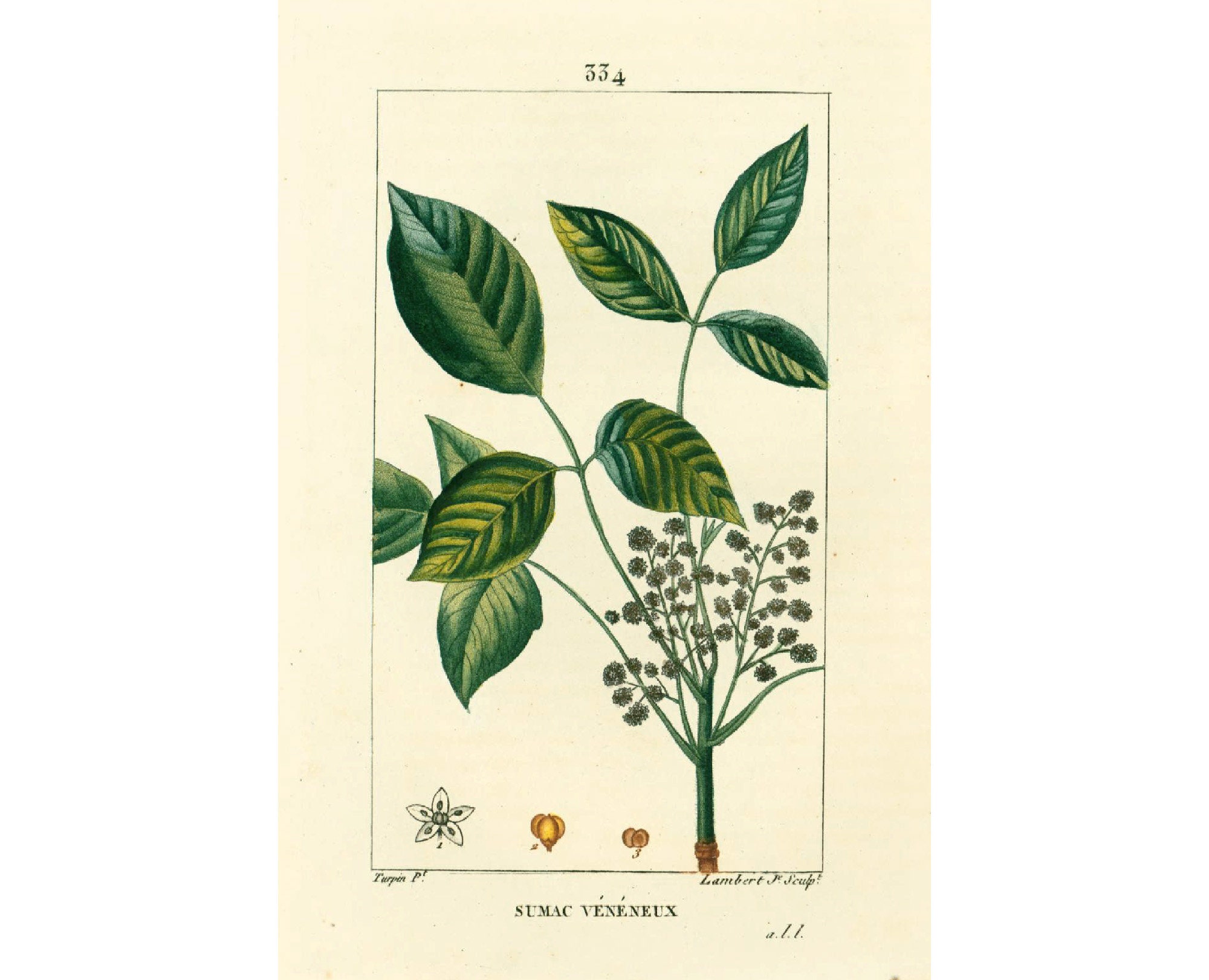The image is of a vintage botanical illustration of a green sumac plant, printed on creamy white paper. The delicate artwork depicts the plant with three main stems, each supporting three green oval leaves shaded with hints of yellow. The main stalk extends shorter twigs bearing small buds and lilac or lavender-shaded flowers, adding intricate detail and highlighting the botanical features. The plant is further adorned with star-shaped images and sketches of its flowers and seed pods. The illustration is encased within a hand-drawn black border and positioned on a crimped background marked with the number 334 at the top. Along the bottom, text identifies the plant as "Sumac Veneneux," though partially obscured. There are additional penned annotations and artistic flourishes, including brown and yellow mustard elements and a black and white flower, enhancing the vintage authenticity of the illustration. The piece is signed by the artist Lambert Desculpt, contributing to its historical charm and botanical significance.